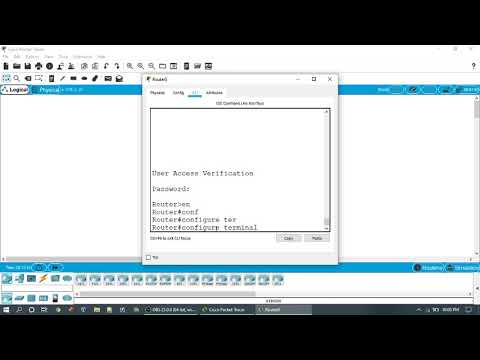This image is a blurry screenshot of a Windows computer screen, framed by thick black borders at the top and bottom. The central focus is a white-background pop-up box with a gray border inside a larger area that also has a white background and is bordered by horizontal blue stripes at the top and bottom. This larger area displays various file icons, suggesting it is part of a computer program, possibly related to networking, given the text and icons visible. Key phrases such as "user access verification," "passwords," "router," "router config," and "router config terminal" appear within the inner pop-up box, which itself has a black border. Additionally, Windows interface elements like the Start menu and clickable buttons (File, View, etc.) are visible in the upper left-hand corner, adding to the detailed documentation of the software displayed. The color scheme includes black, white, off-white, blue, turquoise, gray, and yellow, capturing the essence of the screenshot and the possible networking application in use.